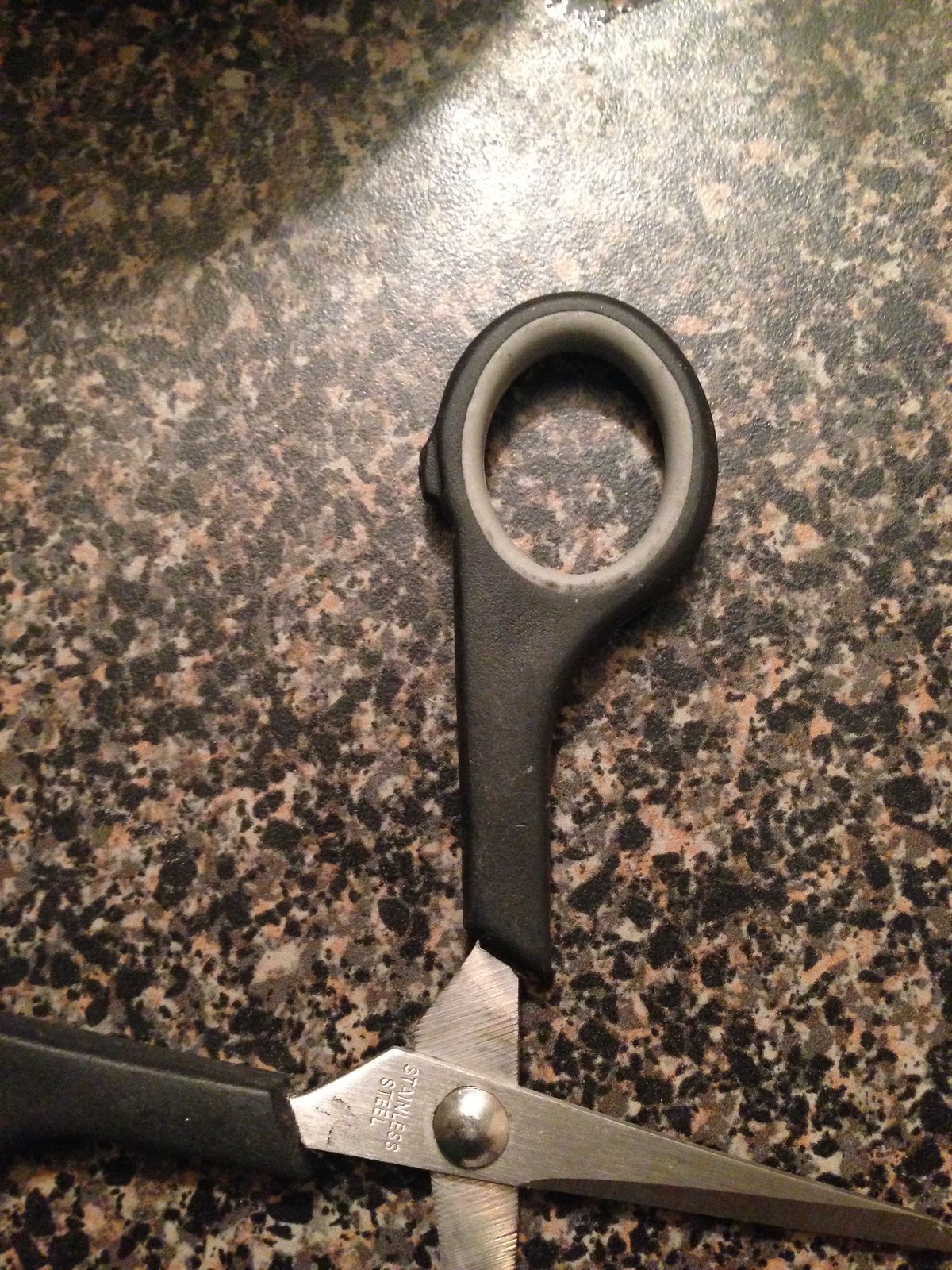This image is a color photograph of a pair of open scissors resting on a glossy granite countertop that fills the entire background. The granite surface exhibits a striking black, white, and reddish-tan marbled pattern with flecks spread throughout. A light source from the upper right illuminates the granite and scissors, casting a shadow in the upper left corner.

The scissors have short, sharp blades, and the partially visible blade has an inscription that is partially legible, reading something akin to "stainless." The handles of the scissors are black with grey-rimmed holes for the fingers. One handle is prominently featured in the middle of the photo, while the other is partially visible, extending towards the bottom left. The visible handle includes a soft, grey rubber grip inside the finger hole. The overall effect is a detailed and well-lit depiction of the scissors against a richly textured stone backdrop.